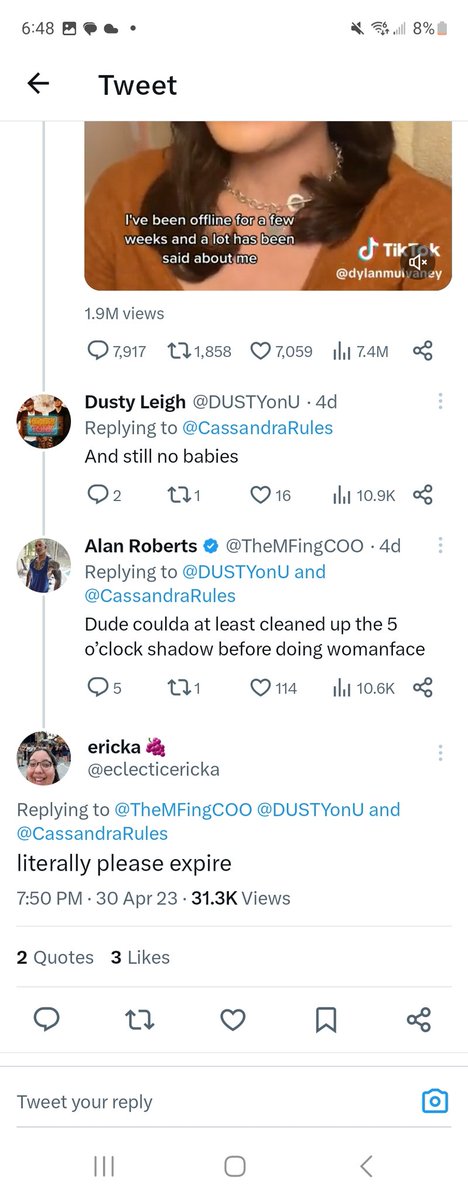The photograph captures a series of tweets prominently featuring a post by Dylan Mulvaney, which reads: "I've been offline for a few weeks and a lot has been said about me." This tweet has amassed significant engagement, with 1.9 million views, 7,917 comments, 1,858 shares, and 7,059 likes.

In the response thread, Dusty Lee (or Dusty Leah) replies to Cassandra Rules with the remark, "and still no babies." Following this, Alan Roberts responds to the discussion with the comment, "dude, could have at least cleaned up the 5 o'clock shadow before doing woman face." Erica then interjects, addressing the previous commenters with the harsh retort, "literally, please expire." This interaction was timestamped at 7:50 PM on April 30, 2023.

Additional engagement metrics include two quoted tweets and three likes on Erica's comment. The interface prompts users to "tweet your reply," inviting further contributions to the conversation. The primary focus of the discourse appears to be Dylan Mulvaney, who, according to the critical comments, is perceived as a man presenting as a woman.